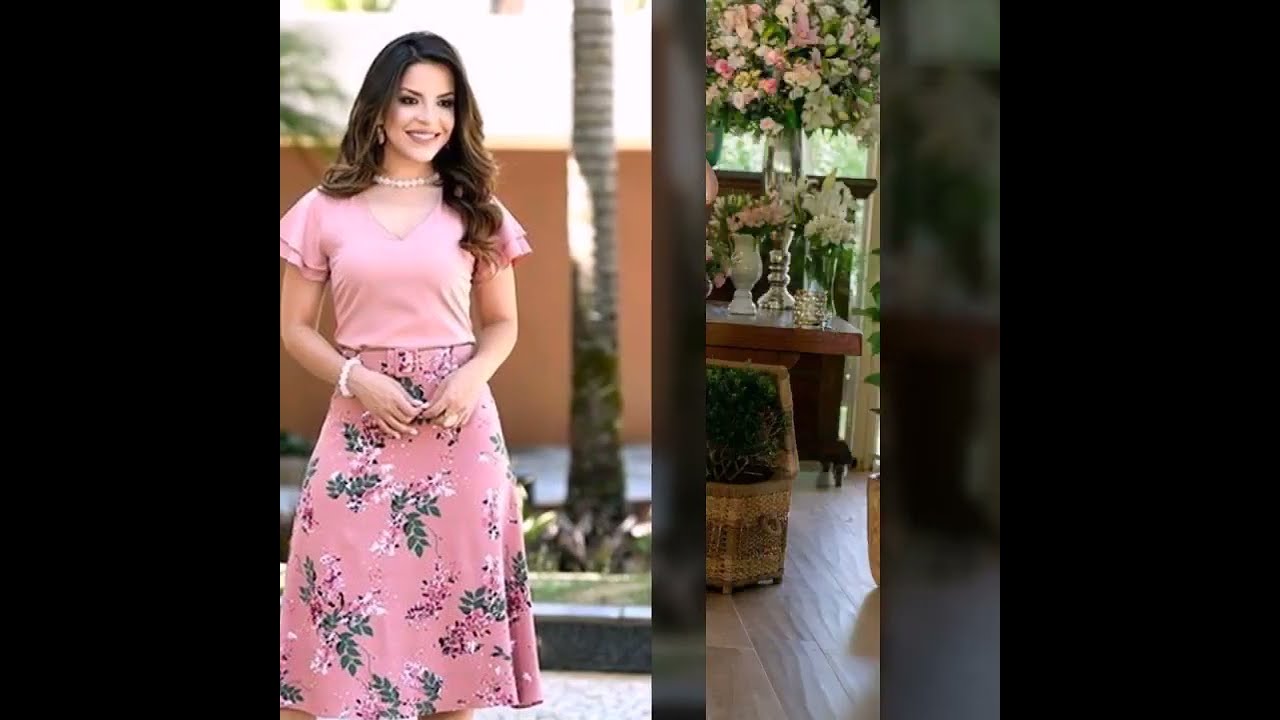The image features a smiling woman with long, dark brown hair streaked with blonde, cascading down her right shoulder. She is adorned in a short-sleeved, pink shirt that falls just below her shoulders, complemented by a matching skirt and belt with green leaf and vine patterns. Her accessories include a white pearl necklace and a white bracelet resting on one wrist. With brown eyes, brown eyebrows, and dark purple lips, she stands with her hands clasped in front of her waist, exuding a graceful presence. In the background on her left, a tree trunk with distinctive rings is visible, while on her right, a wooden floored interior with various vases of flowers rests on top of wooden tables. The scene is an outdoor, professional photoshoot setting, bordered thickly in black.